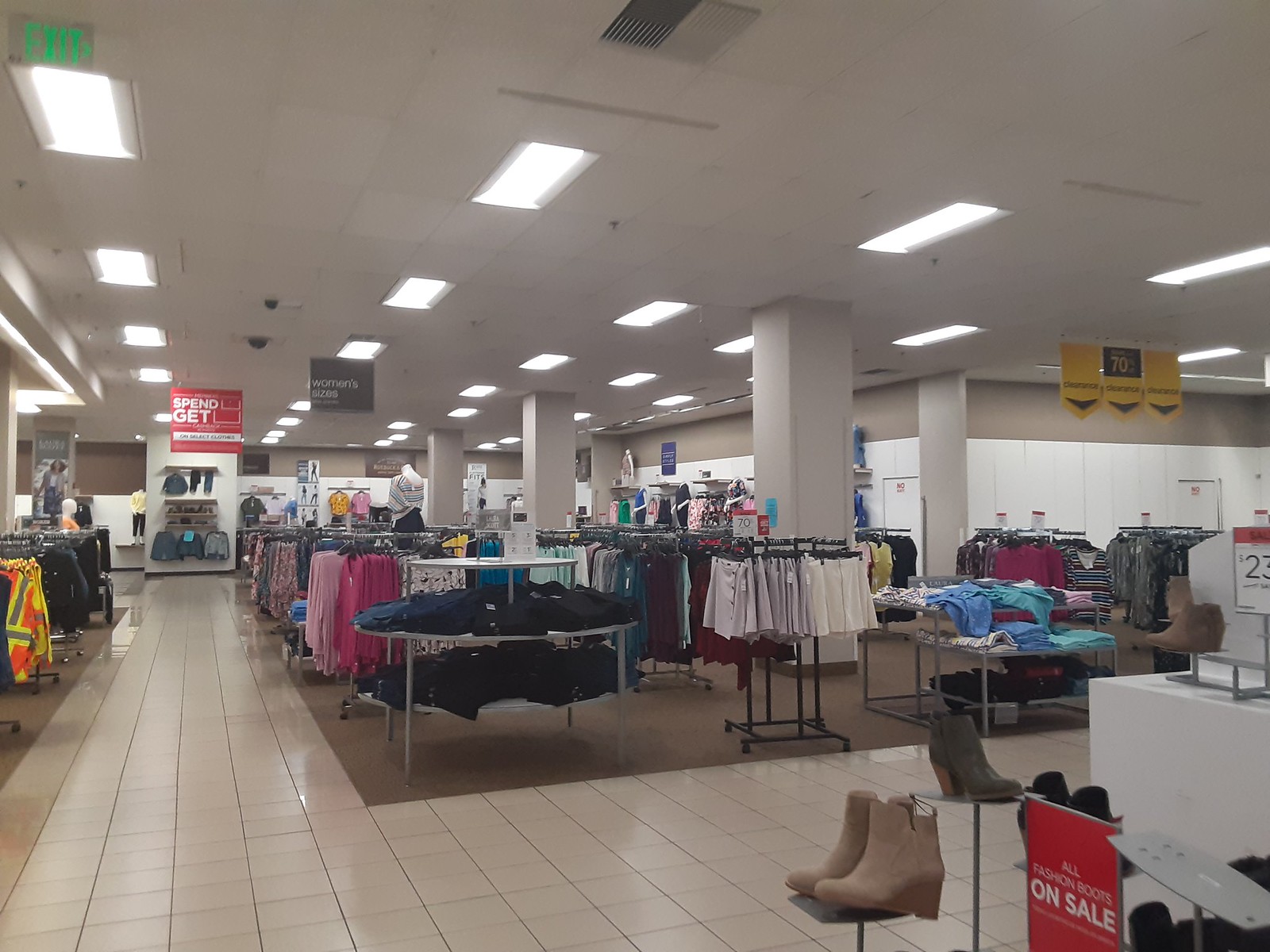The image showcases the interior of a retail clothing store, featuring a typical commercial white ceiling with semi-translucent panels that provide bright, even illumination throughout the space. Clothing in a vast array of colors—ranging from light hues to vibrant reds, blues, and more muted blacks and browns—are neatly arranged on tall steel racks that allow garments to hang and display fully. 

In addition to the hanging clothes, various types of shoes are presented on metal risers and in display cases, creating a focused area for footwear. In the center of the image, a tri-level white table is prominently arranged with neatly folded blue jeans. 

The store's layout contrasts between flooring types; walkways are composed of beige tiles, offering a clean and distinct path for shoppers, while the areas containing clothing are carpeted in brown, providing a softer, more inviting atmosphere. 

Throughout the store, signage is strategically placed, including red signs with white lettering and yellow signs with black text. Notably, there's a large clearance sign visible, indicating a tempting 70% discount on selected items.

Overall, the store presents a well-organized and inviting shopping environment, where careful attention to display and layout enhances the browsing experience.